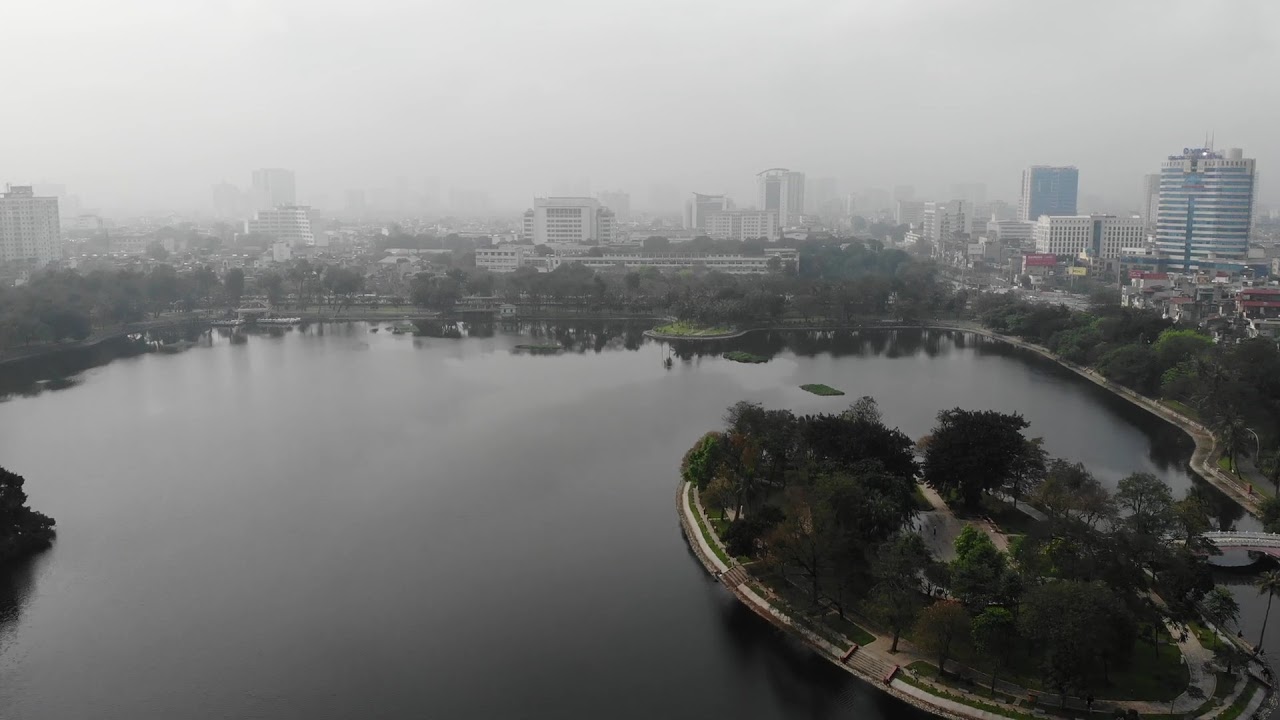The image portrays a sprawling cityscape shrouded in heavy fog and pollution, creating an overall gray, hazy atmosphere. The sky above is a strip of uniform gray, blending seamlessly with the mist that envelops the tops of numerous skyscrapers and buildings. These structures vary in height and width, densely packed together, with some taller buildings obscured by the fog in the background.

In the foreground, starting from the lower part of the image, there is a large body of water, possibly a harbor or pond, reflecting the dull gray of the overcast sky. This water extends from the lower left-hand corner to the middle and right side of the image, appearing murky and dark. Surrounding this body of water, particularly on the right side, is a circular cement area with tall, vibrant green trees.

Further, there's a grassy area lined with dark green trees separating the water from the city’s concrete jungle. The scene is devoid of people on the water, yet faintly visible are a few individuals walking on the cement areas near the trees, emphasizing the contrast between the natural and urban elements of this densely built, polluted cityscape. The image is entirely text-free, capturing a raw, somber snapshot of urban life.